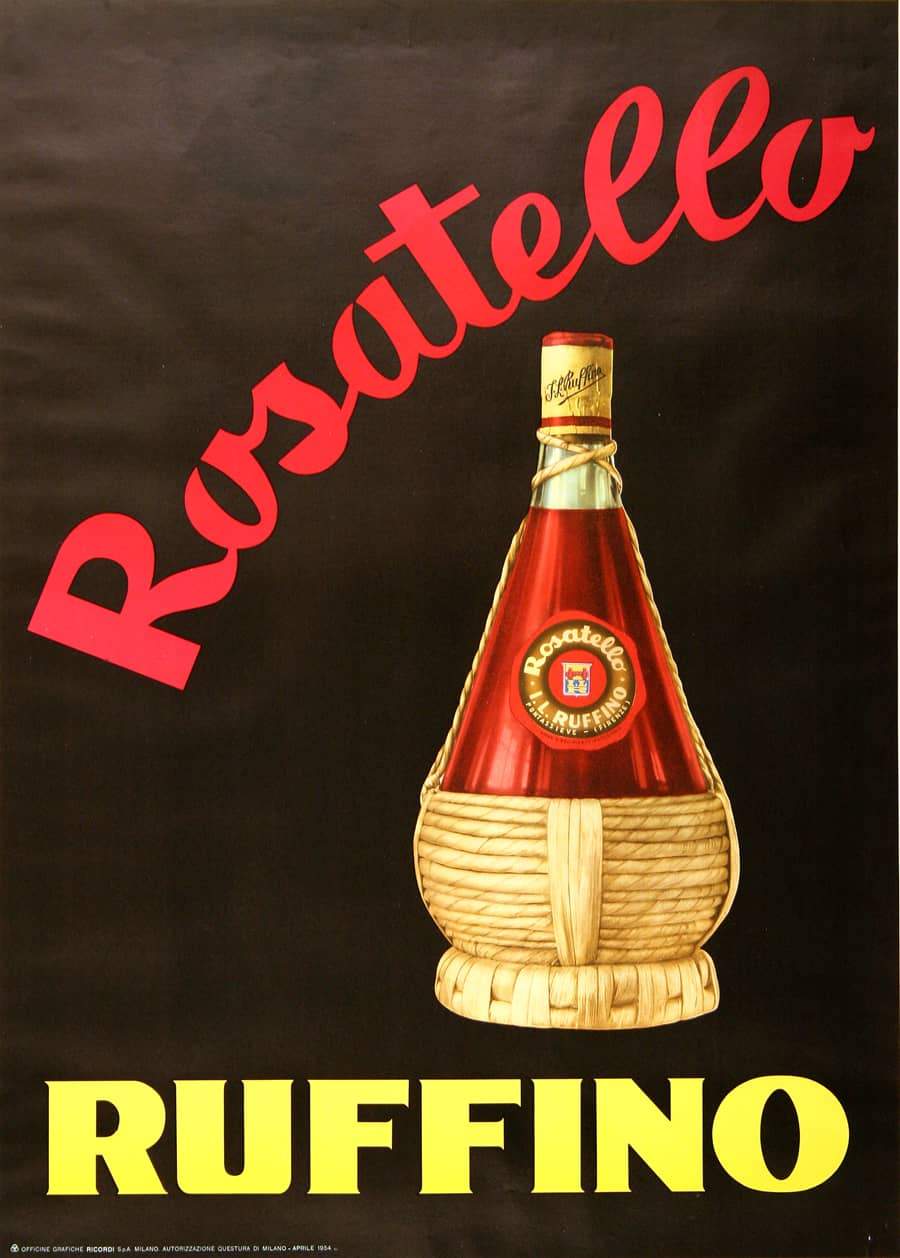The image features a painting of an Italian wine bottle labeled "Rosettelo Rufino." The bottle has a distinctive shape with a slim top that expands downwards and slightly curves. The upper part of the bottle is red, transitioning into brown at the bottom and base. A brown rope-like structure adorns the neck of the bottle, above which the cap, composed of brown and red foil, is situated. At the base, the name "Rosettelo LL Rufino" is displayed in a circular arrangement, with "Rosettelo" in red at the top and "Rufino" in yellow at the bottom. The bottle is nestled in a base made from dried woven leaves, adding a unique touch to its appearance. The background of the image is grey, providing a stark contrast to the bottle's vibrant colors and intricate details.